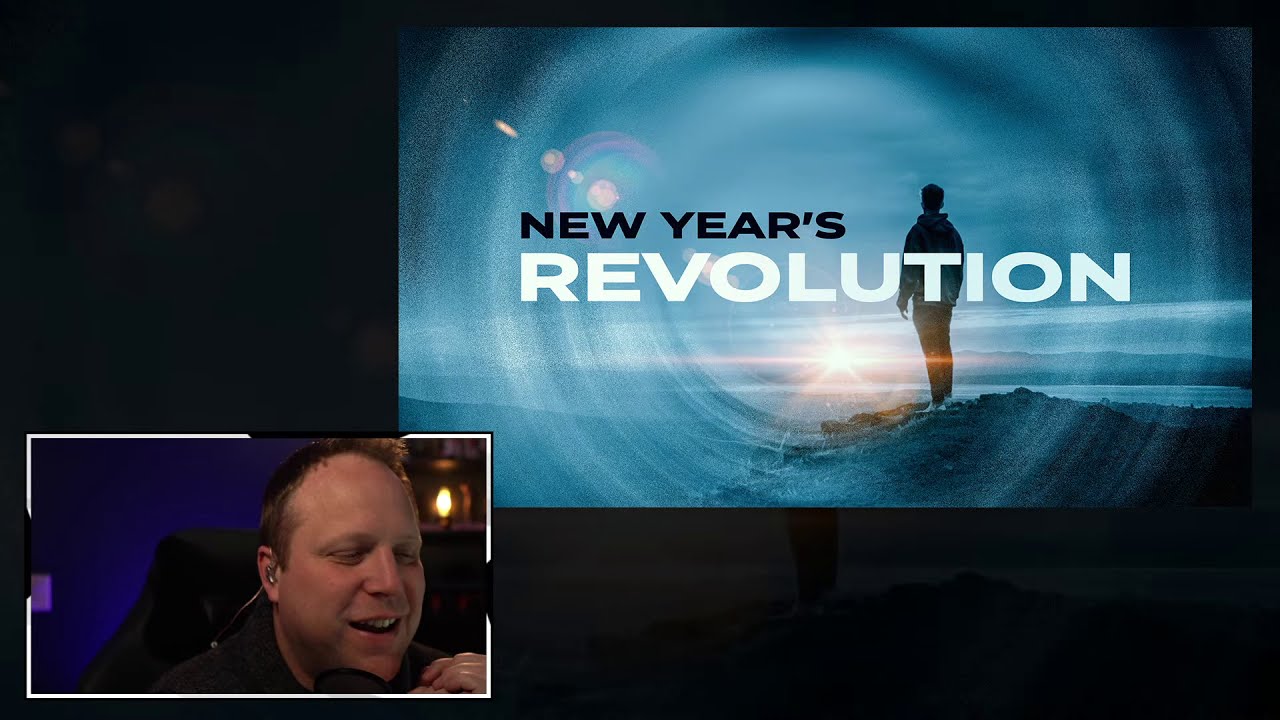The image presents a split-screen scenario with a Caucasian male commentator featured in a rectangular inset on the lower left-hand corner. He is seated, and we can see just the upper part of his shoulders and his head, along with a hint of a black chair behind him. His short yellow hair is visible, and he wears an earpiece while speaking into a microphone. His mouth is open as if he is mid-commentary, and he possibly has a slight smirk on his face, suggesting he finds the content amusing. The background within his inset is purple with a notable yellow light behind him.

Dominating the right side of the screen is an image with the text "New Year's Revolution" in contrasting black and white block print. This text overlays a picture of a man standing on a cliff peak, overlooking a mountain range and possibly some water. The man is facing away from us, slightly off-center, with concentric rings of blue emanating from the sun rising behind him, casting a striking silhouette. The background accompanying the text is solid black, giving a distinct separation from the commentator's inset. The shared perspective suggests that the commentator is actively reviewing or discussing the "New Year's Revolution" scene displayed on the larger screen.